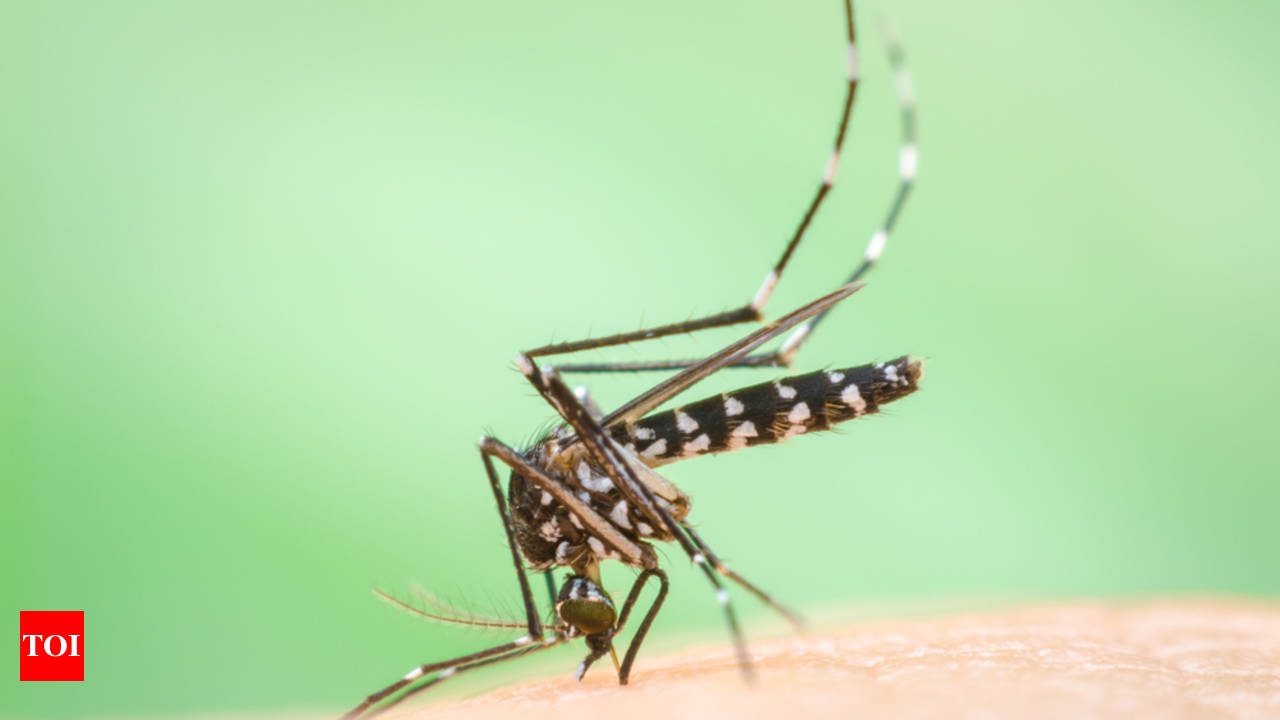This close-up photograph features a mosquito with a dark brown body adorned with white spots and stripes. It is poised with its proboscis inserted into pale skin at the bottom of the image. The background is a mint green with areas that fade into lighter shades, almost white, primarily in the middle and off to the right. In the lower left corner, there is a small, bright red square with uppercase white letters that appear to read "T-O-I". The mosquito's slender legs and long, flat back are clearly visible, highlighting the intricate details of its anatomy.